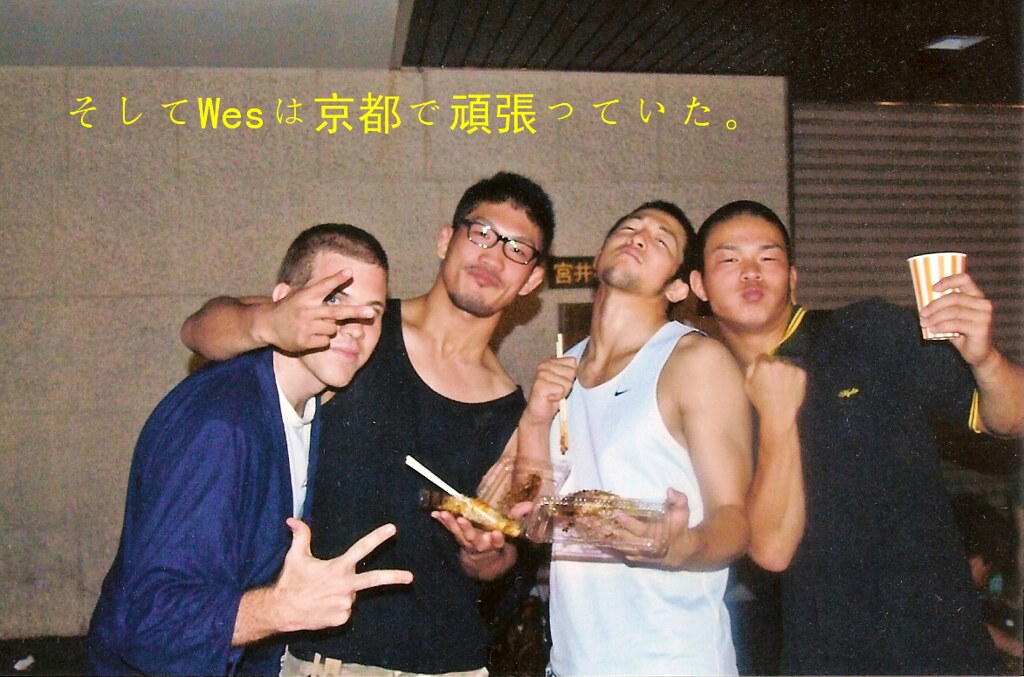In this vibrant photograph, four young men, enjoying each other's company, are captured standing closely together, each contributing to the lively atmosphere. The young man on the far left, who appears to be white, is wearing a blue dress-like shirt over a white t-shirt and is playfully giving a peace sign with his right hand. His gesture overlaps with the face of the young man next to him, who is of Asian descent, wearing a black t-shirt and black glasses. This second gentleman also has his right hand up in a peace sign, while his left hand holds a plastic container, possibly containing chicken, with chopsticks sticking out. The third young man, also Asian, is adorned in a white tank top with a small black Nike logo. He is seen holding a similar plastic container of food, immersed in his meal with chopsticks in his right hand. His expression suggests he is savoring something delicious. The fourth individual, positioned on the far right, is another Asian gentleman clad in a black t-shirt with yellow trims. He exhibits a look of accomplishment while raising his left fist and holding a white and orange vertically striped paper cup. Adding to the cultural context, there is a Mandarin caption in the top left corner of the image. The interconnected poses and shared gestures among these young men create a snapshot of camaraderie and joy.